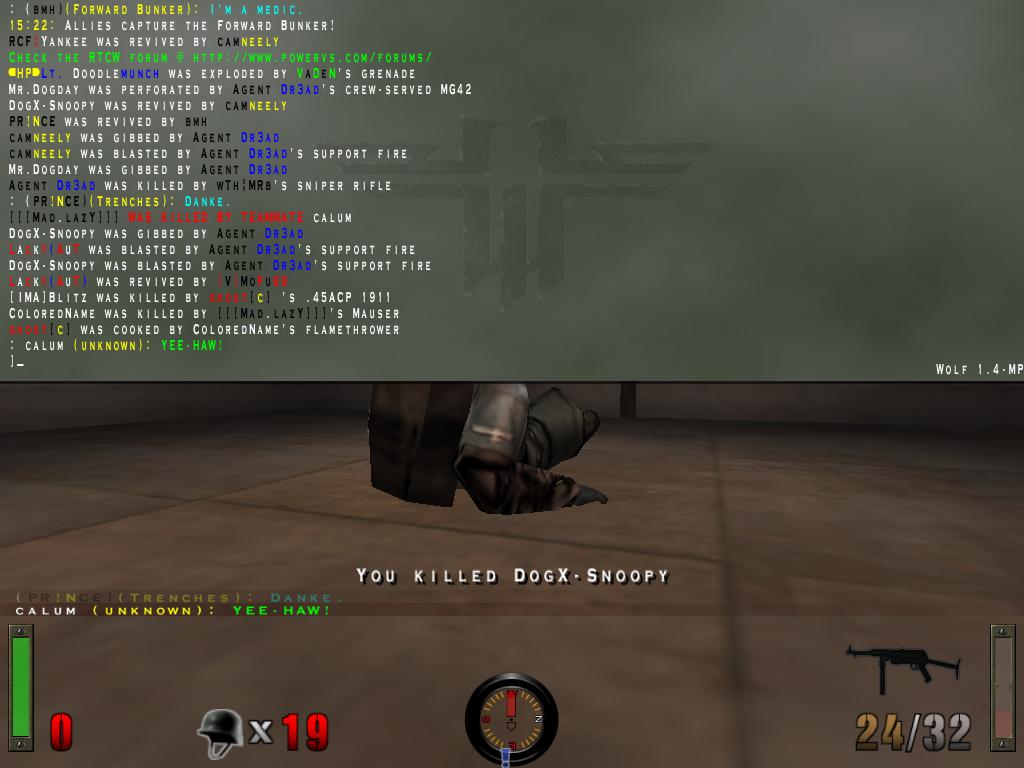Screenshot from a video game depicting a significant event. The image is dense with text, indicating critical in-game information. Prominently, there is an announcement stating, "Allies capture the forward bunker," suggesting a pivotal moment in the gameplay. The player's role appears to be a medic, highlighting their supportive function in the game. Another line mentions "Yankee was received" and directs the player to "Check the RCTW," likely instructions related to the immediate game objectives. The foreground displays an attempt counter, showing "24 to 32 attempts," while another note mentions the player killing an enemy identified as "dog X Snoopy." It appears to be the initiation phase of a mission or level within the game, setting the stage for forthcoming actions.